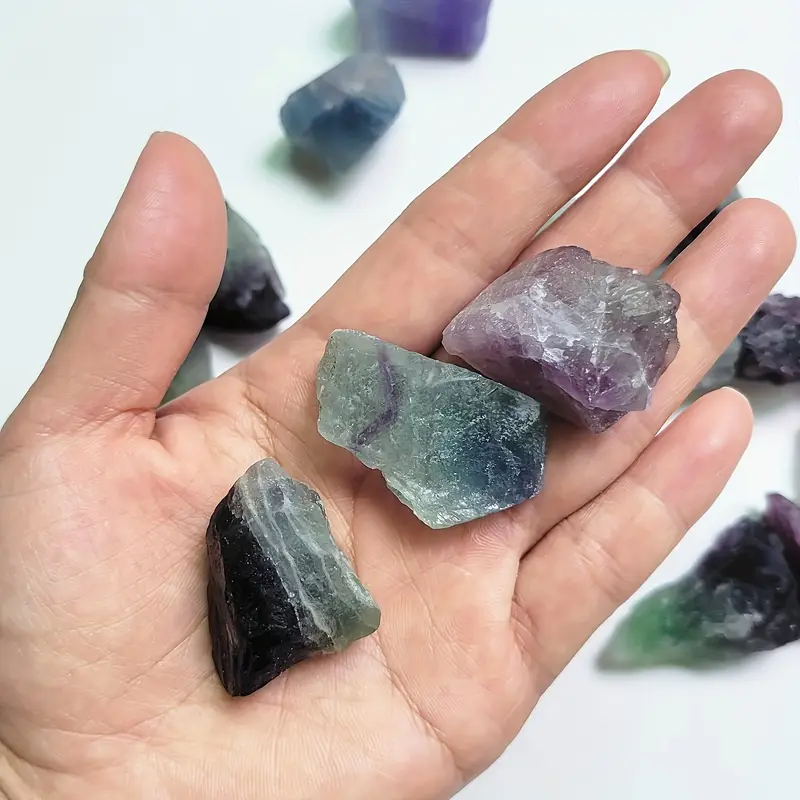A photograph showcases an individual's open left hand, visually centered in the frame, holding three distinct, unpolished gemstones. These rocks, which exhibit gem-like colors and textures, appear to be rough minerals, potentially quartz or other special stones. The top gemstone in the person's palm is a deep, translucent purple, catching the light from various angles. The middle rock has an intriguing combination of green and light purple, almost translucent with a striking purple stripe through it. The bottom gemstone is predominantly black with dark gray tones and interspersed white lines, creating a banded appearance. Surrounding the hand, the slightly blurred background reveals an assortment of other colorful, scattered rocks on a white surface, suggestive of a collection of special stones.